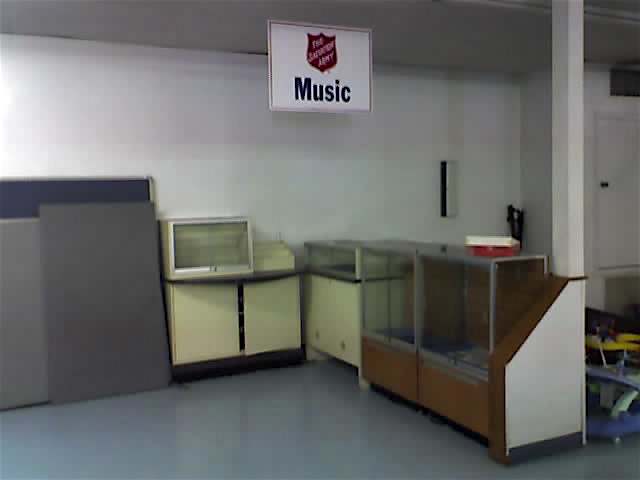In this image, we are viewing an empty section within a Salvation Army store, once dedicated to selling music. Suspended from the ceiling is a white sign confirming this previous use. The store has a clean, shiny gray floor that reflects the light. There are several empty display cases, each distinct in color and style: a dark brown case with square glass panels, two cream-colored cases, a smaller case placed above, and a large gray case. Behind these display cases, baby equipment of various colors, including yellow and purple, is visible. The background features a cinder block wall painted white, adding to the stark, clean appearance of the space.